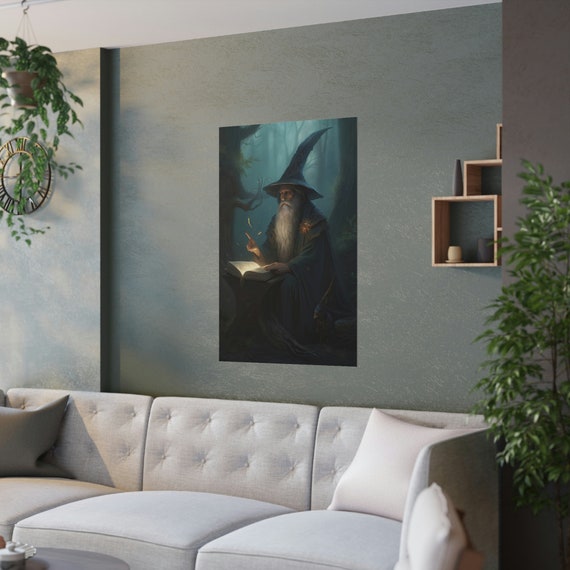The image depicts a cozy living room with a cream-colored couch adorned with two decorative pillows—one on each end. Behind the couch, the wall is painted a grayish-green hue and prominently features a dark, moody painting of a wizard. The wizard, who resembles Dumbledore with his long beard and tall, slightly curved hat, is seated in a forest, gazing intently at an illuminated book on his lap. To the right of the couch stands a tall house plant, adding a touch of greenery to the room. Above the couch on the left side, a hanging plant partially obscures a metal clock with Roman numerals, which has no glass and is see-through. Below the clock, barely visible, is a small portion of a coffee table with a few items on it. The overall decor of the room, complete with wooden cubbies on the right wall (partially visible due to the angle), exudes a warm and inviting atmosphere that could be straight out of a lifestyle catalog.